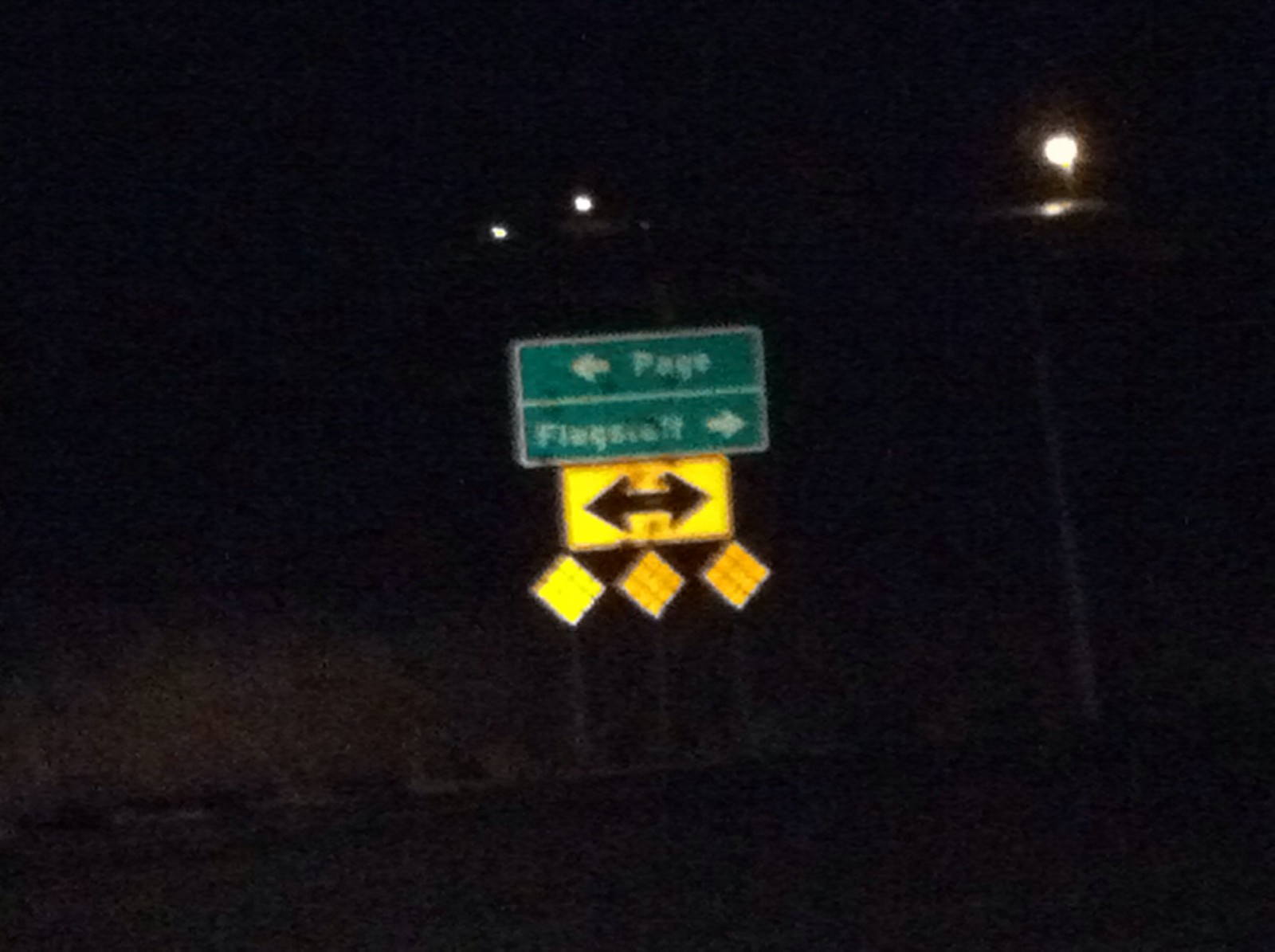The image, taken from a first-person point of view at nighttime, captures a street sign on a dimly lit road. The surroundings are pitch black, with the illumination provided by three visible street lamps—one on the right side of the image and two further in the distance behind the main focus of the photograph. The signage, held up by three large poles, consists of multiple components: 

1. At the top, a green rectangular sign is split into two sections. The left section reads "PAGE" with a white arrow pointing left, while the right section indicates "FLAGSTAFF" with a white arrow pointing right.
2. Below the green sign, there is a yellow rectangular sign with black arrows pointing both left and right, highly reflective under the light from what appears to be the camera or headlamps of a car.
3. Further down, arranged in a diamond shape, are three yellow reflective signs.

The bright reflections from the signs' surfaces are prominent against the dark backdrop, enhancing their visibility in the night setting.